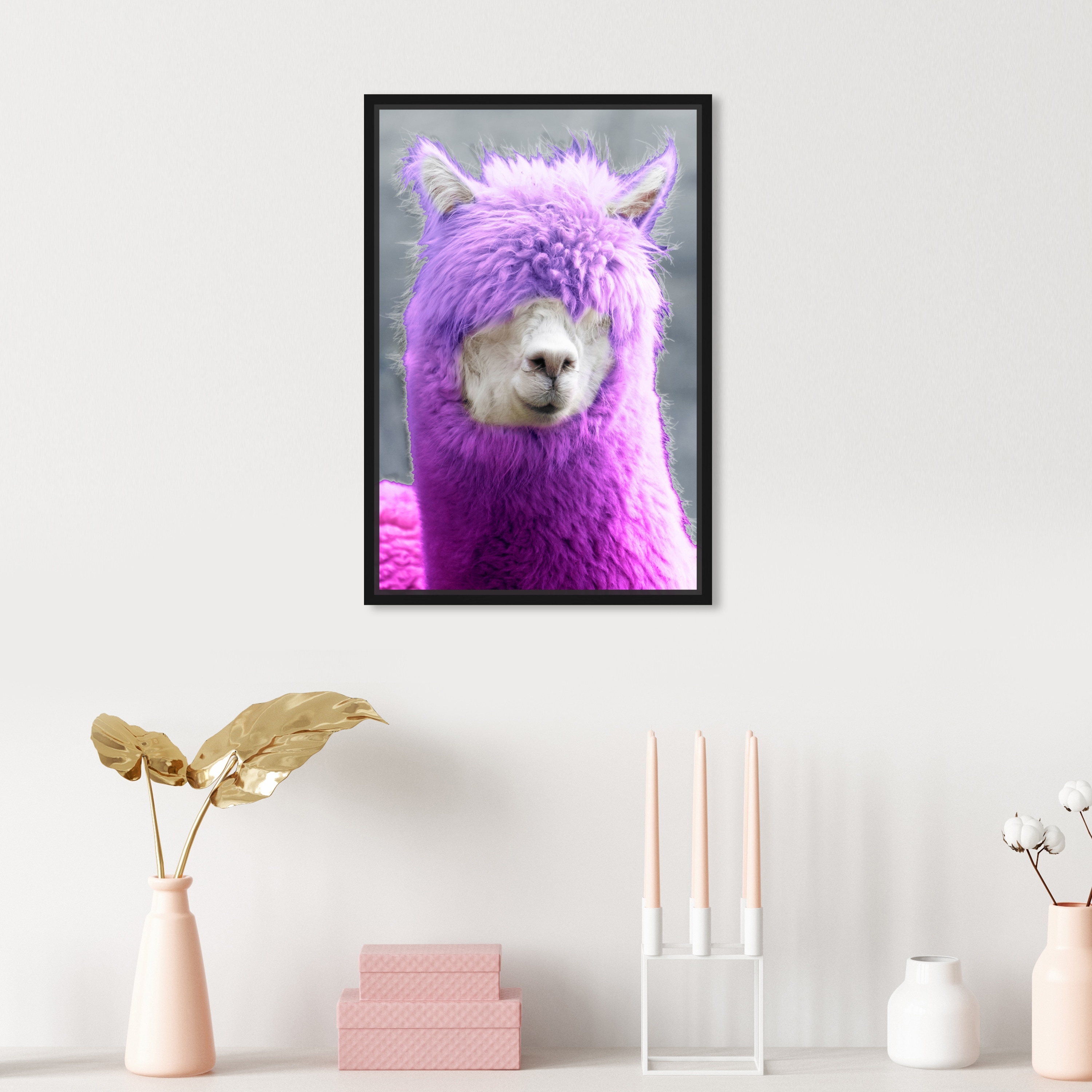The image showcases a framed picture on a plain white wall. The picture, surrounded by a black frame, features a llama or alpaca with a striking appearance: it has a fluffy, purple mane that covers its eyes, leaving its white muzzle and the white insides of its pointy ears visible. The background of the framed picture is gray. Below this picture, on an elevated white surface such as a table or shelf, there's an arrangement of items. A beige vase holds golden philodendron leaves that look metallic. Next to the vase are two small pinkish off-white boxes stacked on top of each other, adorned with faint white stripes. Further to the right is a clear candle holder, trimmed in white, containing three thin, long off-white candles. Completing the display are two pottery vases; the off-white pink vase is taller and has cotton stems protruding from it, while the shorter white vase stands empty.